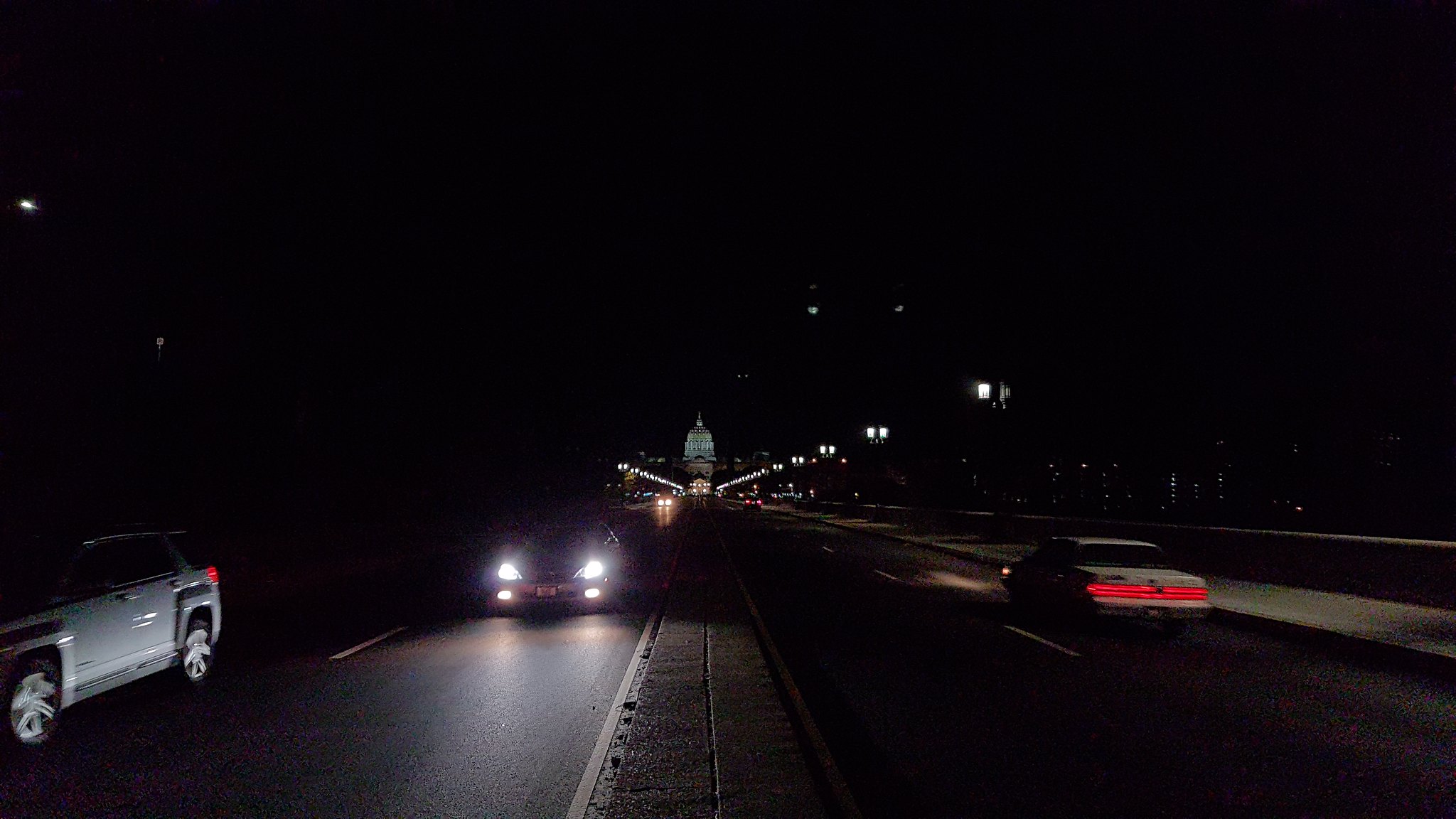The image captures a bustling urban street at night, featuring two roads, each encompassing two lanes. The road on the left exhibits oncoming traffic, while the road on the right carries vehicles moving away from the viewer towards a dimly lit, distant building with an illuminated dome, resembling a city's capitol building. The nocturnal scene is adorned with street lamps positioned on both sides of the road, with those on the right more prominently visible halfway down the street.

On the right side of the image, a sedan is observed with its brake lights glowing red. To the left, a white SUV is seen, partially out of the frame, accompanied by another sedan with bright white headlights approaching. Additional vehicles are discernible in the distance, navigating towards and away from the illuminated dome, adding a dynamic liveliness to the nighttime cityscape.